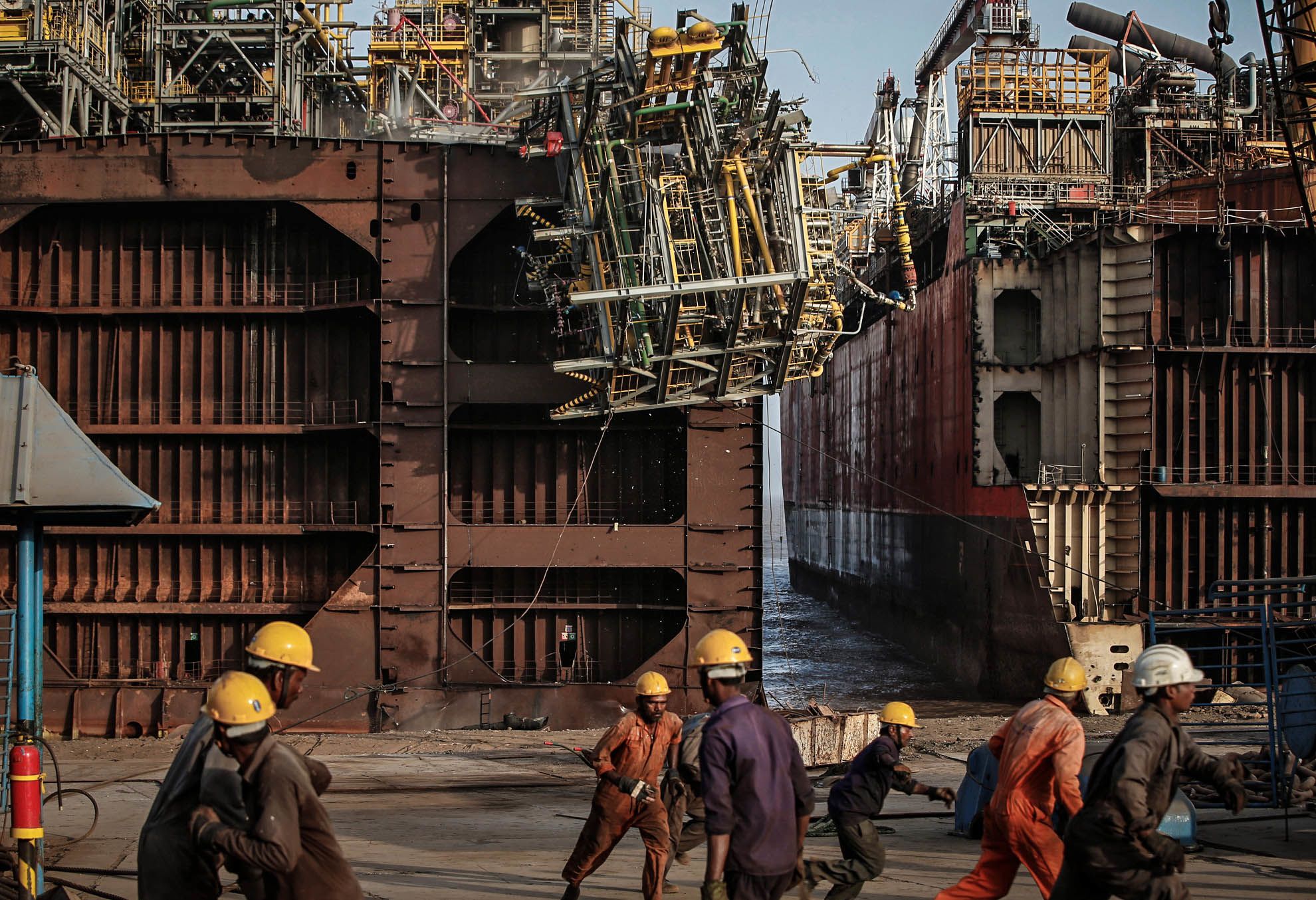The photograph captures a chaotic moment at a bustling shipyard, where two massive freight ships are docked. On the left side, a dark brown shipping container partially obstructs the view of one ship, while a red ship with dark brown accents is docked on the right. In the foreground, seven workers are seen running in various directions, clearly alarmed. Six of the workers, who are mostly moving to the right or towards the camera, are wearing yellow hard hats, while the figure on the far right sports a white hard hat. Their jumpsuits vary in color: two in purple, two in orange, one in brown, one in gray, and one in black. The sense of urgency and fear is palpable as a large, precariously hanging metal structure of tubes and wires looms overhead, appearing to have broken free from the top of the shipping container behind them, posing an imminent danger.